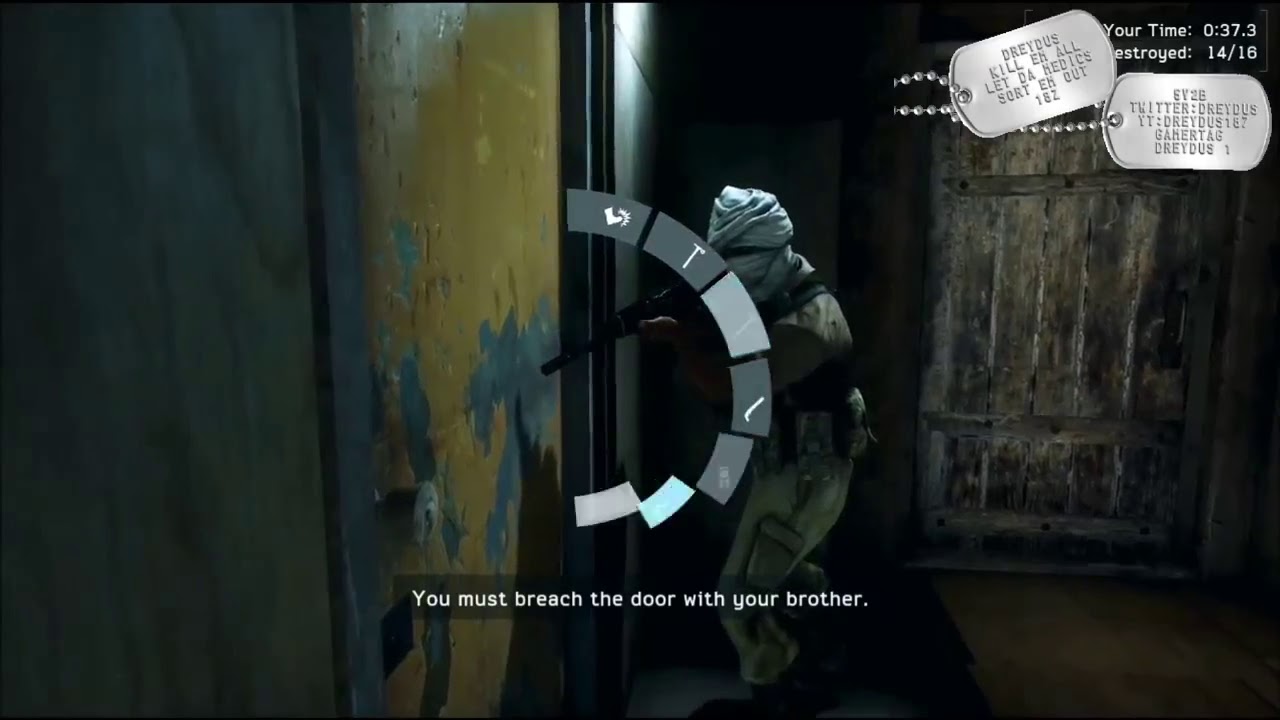This is a horizontal rectangular screenshot from a video game. The central focal point of the image is a character facing left, clad in a brownish-gray camouflaged armor uniform with a gray scarf or turban completely covering their face, leaving just a slit for the eyes visible. The character holds a black machine gun pointed at a stone wall on the left side of the image. The wall features a door, and there is an on-screen prompt below reading "you must breach the door with your brother" in white text. In front of the character is a series of small curved rectangles, likely representing interactive options, one displaying a boot and another a hammer. In the upper right-hand corner, there are two silver dog tags with inscriptions: one reads "Dratus. Kill them all. Let Dratus sort them out. 182," and the other says "Twitter Dratus. Dratus 162. Gamer tag Dratus." The right side of the image showcases a large wooden door made of vertical strips with horizontal slats, set against a wooden floor visible at the bottom. Additionally, the top right shows the end of the word "destroyed," partially obscured by the dog tags, as well as a time of 037.3 and a numerical sequence "14/16."